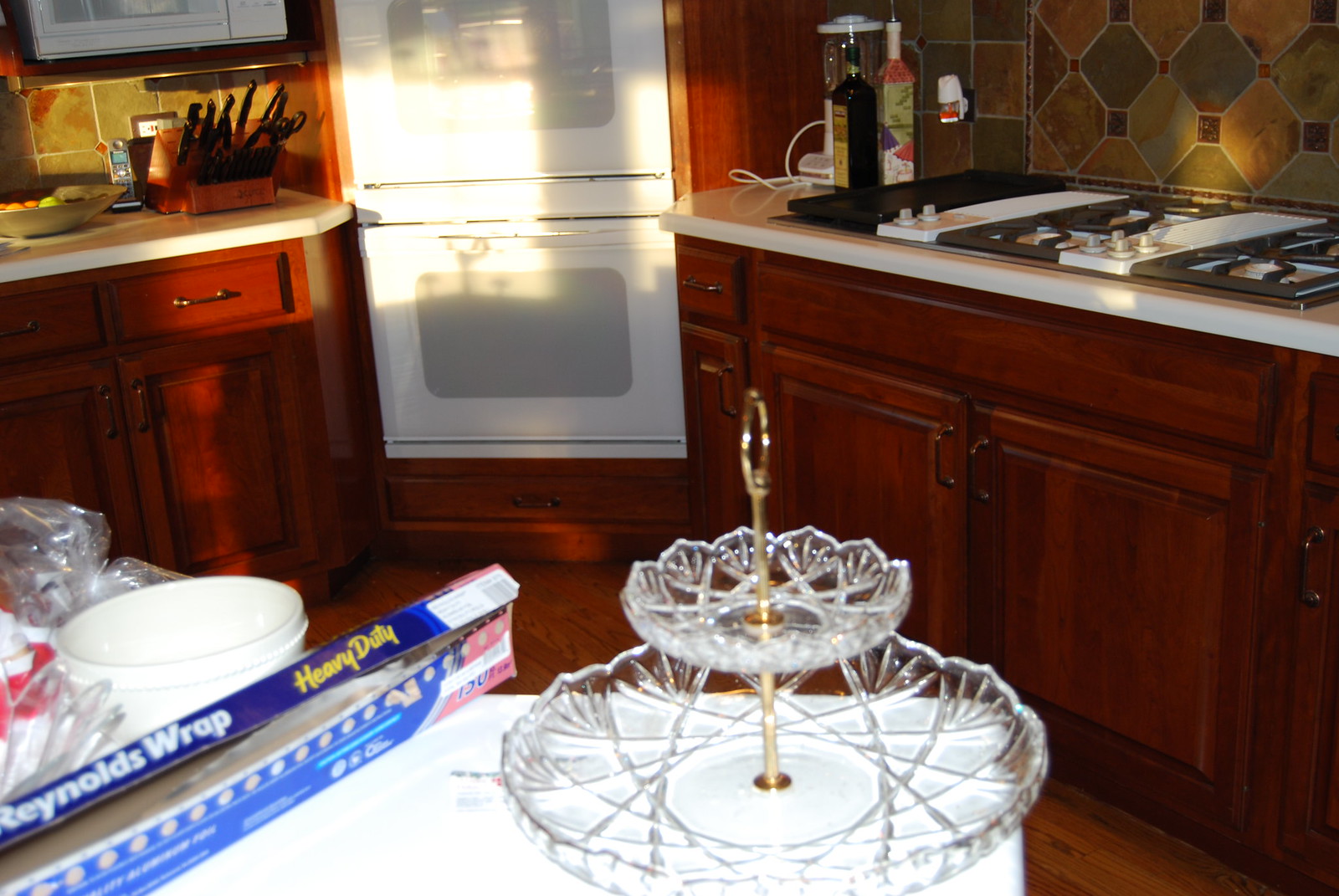The color snapshot captures a cozy kitchen bathed in sunlight flooding through a window on the opposite side of the room, illuminating the entire space with a warm, inviting glow. Of particular interest in this photograph is a pair of white wall ovens, one stacked atop the other, installed into an unusual corner location. These ovens catch and reflect the sunlight, making them appear brilliantly sunny.

Surrounding the ovens are reddish-brown cabinetry, adding a touch of rustic charm to the setting. The cabinetry meets at the corner where the ovens are situated, each side complemented by a set of base cabinets. The countertop adorning these cabinets is a thin, solid surface in a white or light color, hinting at a sleek, modern design.

The backsplash, adding a splash of color and geometric interest, features an intriguing pattern of olive green, tan, and yellow diamond shapes interspersed with small dark brown squares. To the right of the photo, a gas cooktop with white dials and controls stands out, indicating functionality and convenience. Near the cooktop, a couple of bottles, likely containing olive oil and another cooking ingredient, are placed for easy access. An essential oil plug-in air freshener hints at the presence of comforting aromas wafting through the space.

Beside the double ovens, a knife block filled with knives and scissors can be seen, with a microwave mounted above it, adding to the kitchen's efficiency. In the foreground, the corner of a white table is visible, adorned with a two-tiered candy dish made of crystal or glass, adding a touch of elegance. Nearby, a roll of Reynolds Wrap heavy-duty foil and a couple of white balls rest on the table, suggesting ongoing kitchen activity.

The overall scene is an inviting blend of functionality and warmth, with thoughtful details and sunlit charm making it a delightful kitchen snapshot.